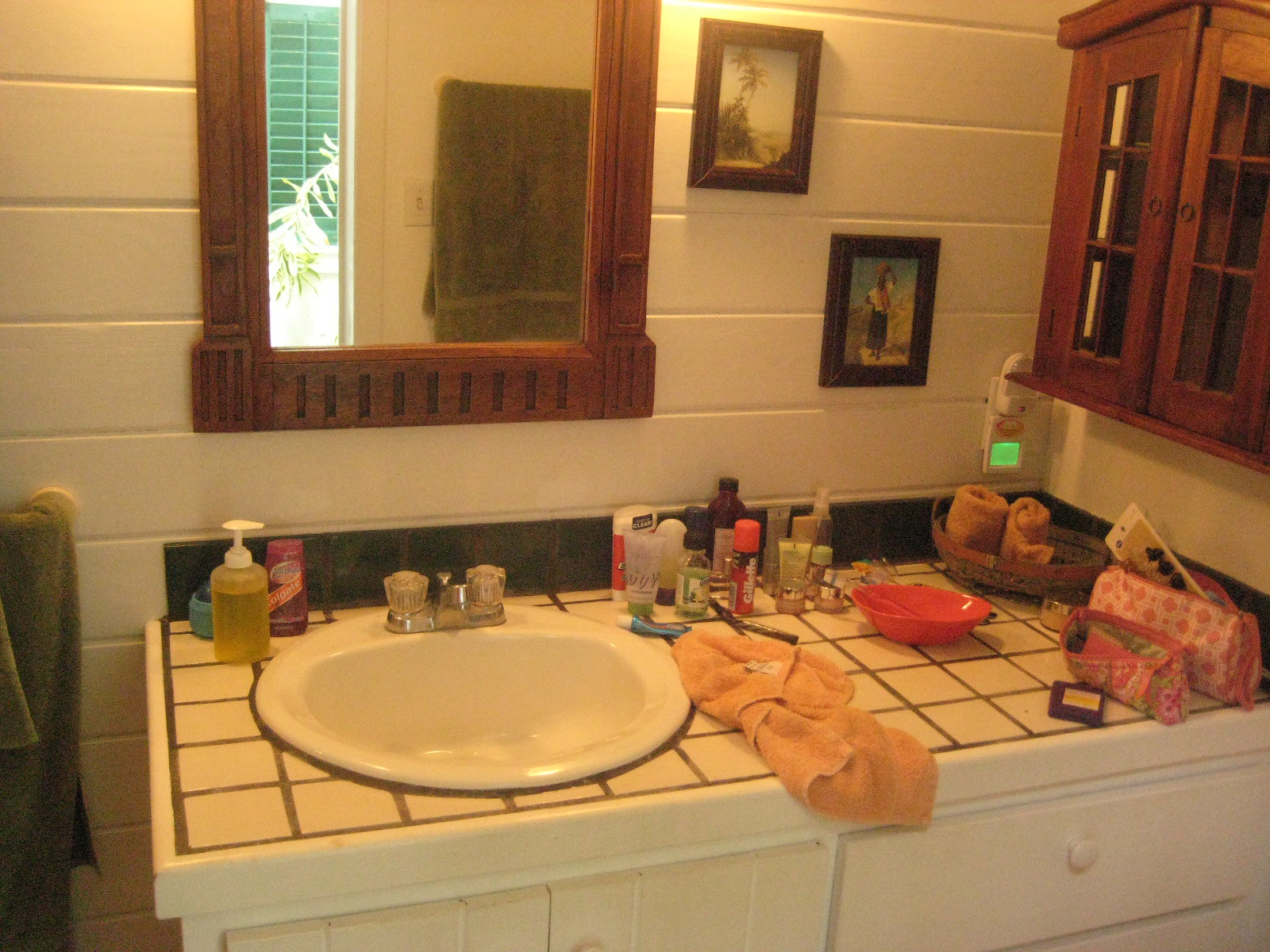A cosy bathroom adorned with light beige concrete block walls provides a serene atmosphere. A green towel hangs neatly on a rack, casting its reflection in a centrally positioned mirror encased in a rustic round wooden frame. To the right of the mirror, a light switch is visible, along with a glimpse of the shower curtain bearing a design of a large white flower with green leaves.

Flanking the mirror are two small framed pictures, adding a touch of personal charm. At the end of the wall stands a white cabinet, featuring two doors with glass panels and a set of drawers on the right side. The cabinet rests on a countertop decorated in a light beige checkerboard pattern with darker beige accents.

The bathroom features a rounded sink equipped with silver faucets and clear white handles. Atop the sink, a pink deodorant, a yellow pump soap dispenser, and a little blue jar are arranged alongside several makeup tubes. A small pink bottle with a pink cap, a brown bottle, a pink bowl, and additional beauty products contribute to the clutter.

Below the counter, a basket containing two rolled washcloths is placed next to two pink printed makeup bags, completing the charming and functional space.